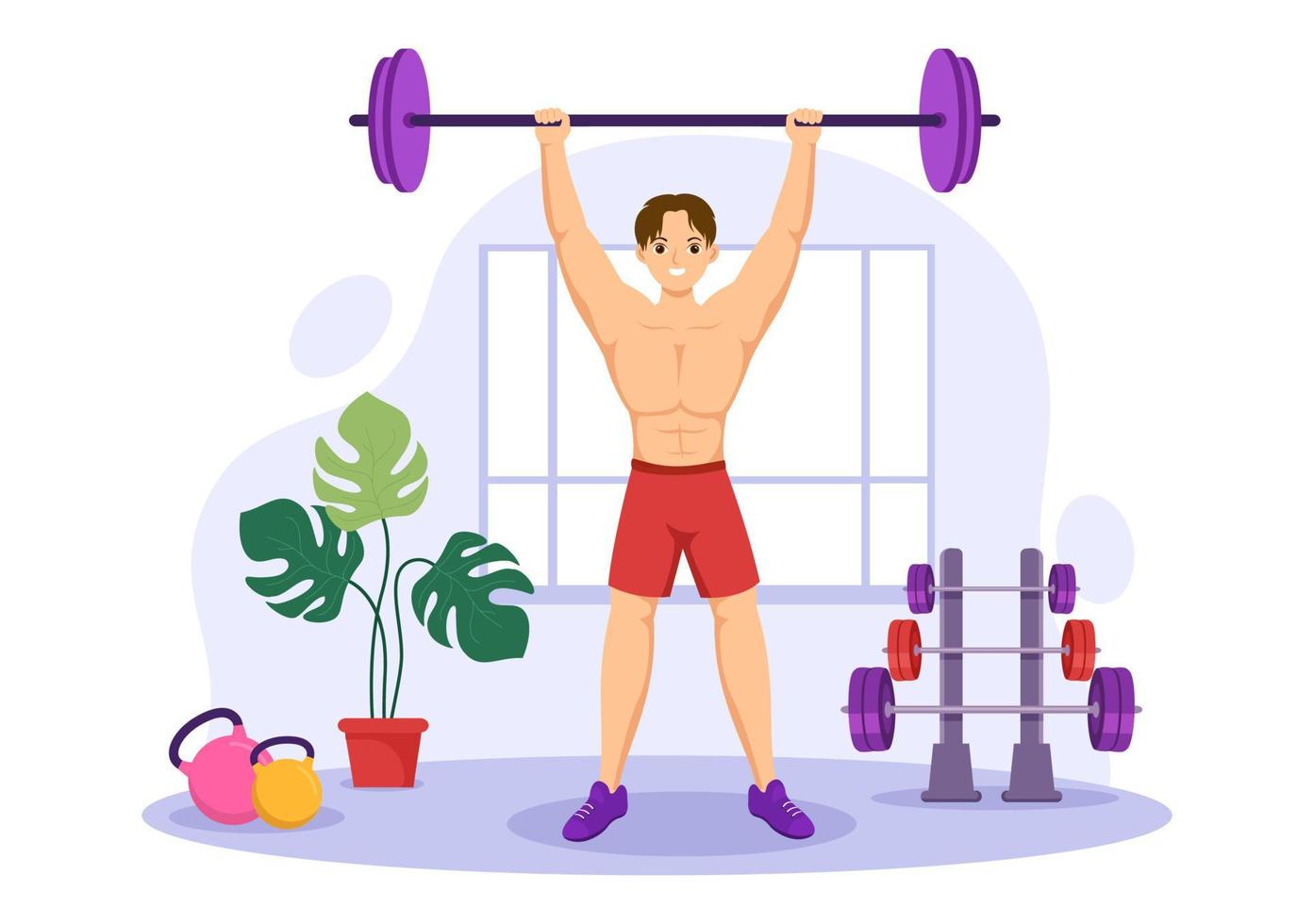The illustration depicts a strong, shirtless cartoon boy, confidently smiling as he holds a barbell with purple weights over his head. He has brown hair and dark eyes, and wears red shorts and purple shoes. He stands in front of a blue-framed window against a white background, with an oval light blue pattern below him. To his left is a houseplant in a burnt orange pot with three large leaves: the outer two being dark green and the middle one lighter green. Next to the plant are two kettlebells; the larger one is pink with a black handle, and the smaller is yellow, also with a black handle. Further to his left, a rack holds a set of three dumbbells: the smallest with purple weights, the medium with red weights, and the largest on the bottom tier again with purple weights. The image is colorful with a strong emphasis on purple, portraying a lively workout scene.